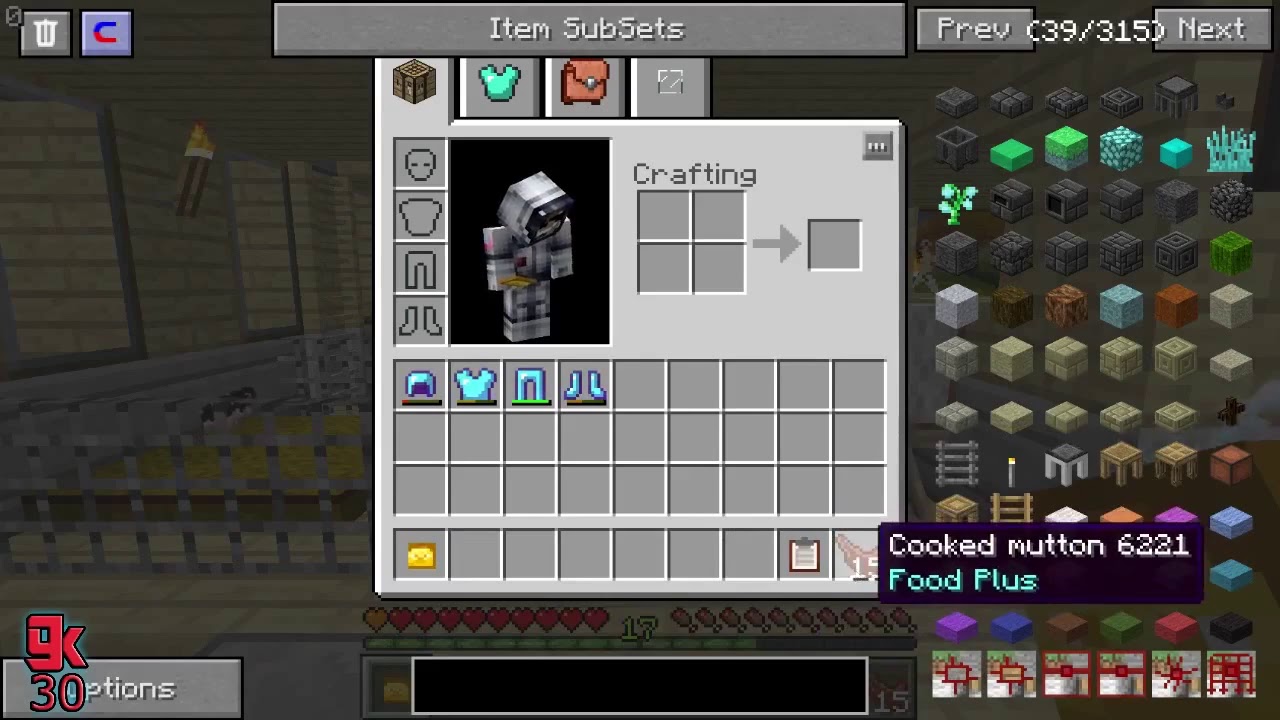This detailed screenshot from the popular video game Minecraft showcases the game's distinct blocky, pixelated graphics. Dominating the image is the in-game inventory screen, placed centrally, clearly displaying the player's selections: several pieces of blue and purple armor equipped on the character. The grey user interface (UI) buttons are aligned at the top, providing various interactive options, including 'Item Subsets' and 'Preview C39'. On the right side, the screen features an array of potential building blocks and items categorized for selection, including boxes, stools, and other crafting components, with labels such as "Cooked Mutton 62" and "Food Plus". The search bar, located at the bottom, is black, facilitating quick item searches. Moreover, a grey 'Options' button is positioned at the bottom left corner adjacent to a '9k 30' label. This meticulous setup suggests the player, possibly identified as TK30, is engaged in organizing and selecting items, perhaps preparing for a building project or game setup, highlighting the rich, intricate inventory management system within Minecraft.